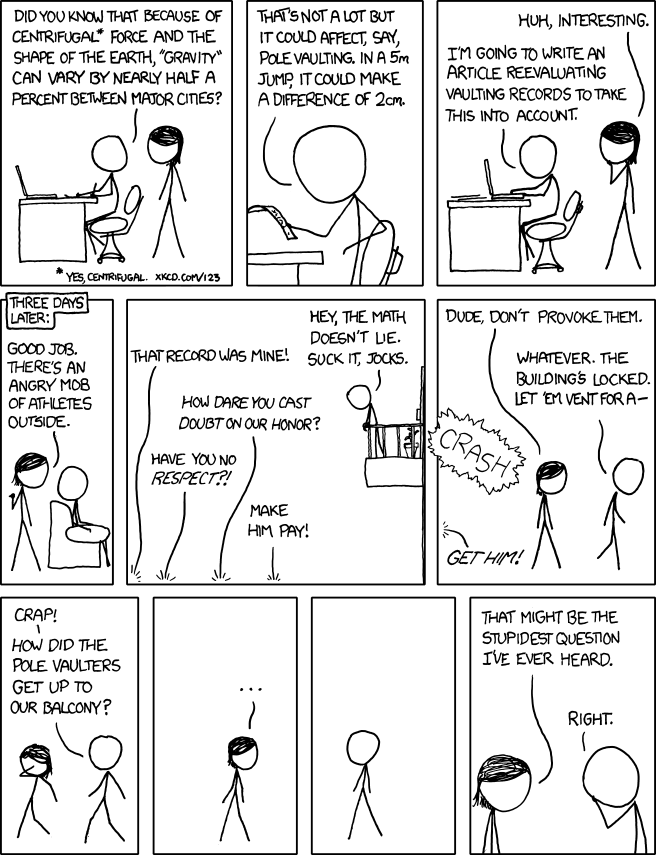"An interesting fact about the Earth's shape and centrifugal force: Did you know that gravity can vary by nearly half a percent between major cities? Although this difference is small, it could affect athletic performances like pole vaulting over a 5-meter bar, potentially causing a variance of about two centimeters. An article highlighted that very few records take this into consideration, which caused quite a stir. Imagine a scene where an angry mob of athletes, feeling their records are being doubted, confront a group inside a locked building. The athletes might attempt to pole vault up to a balcony in frustration. Amidst the chaos and the crash, desks are overturned, and the commotion emphasizes the dramatic clash between science, athletic pride, and the humorous exaggeration of the situation."